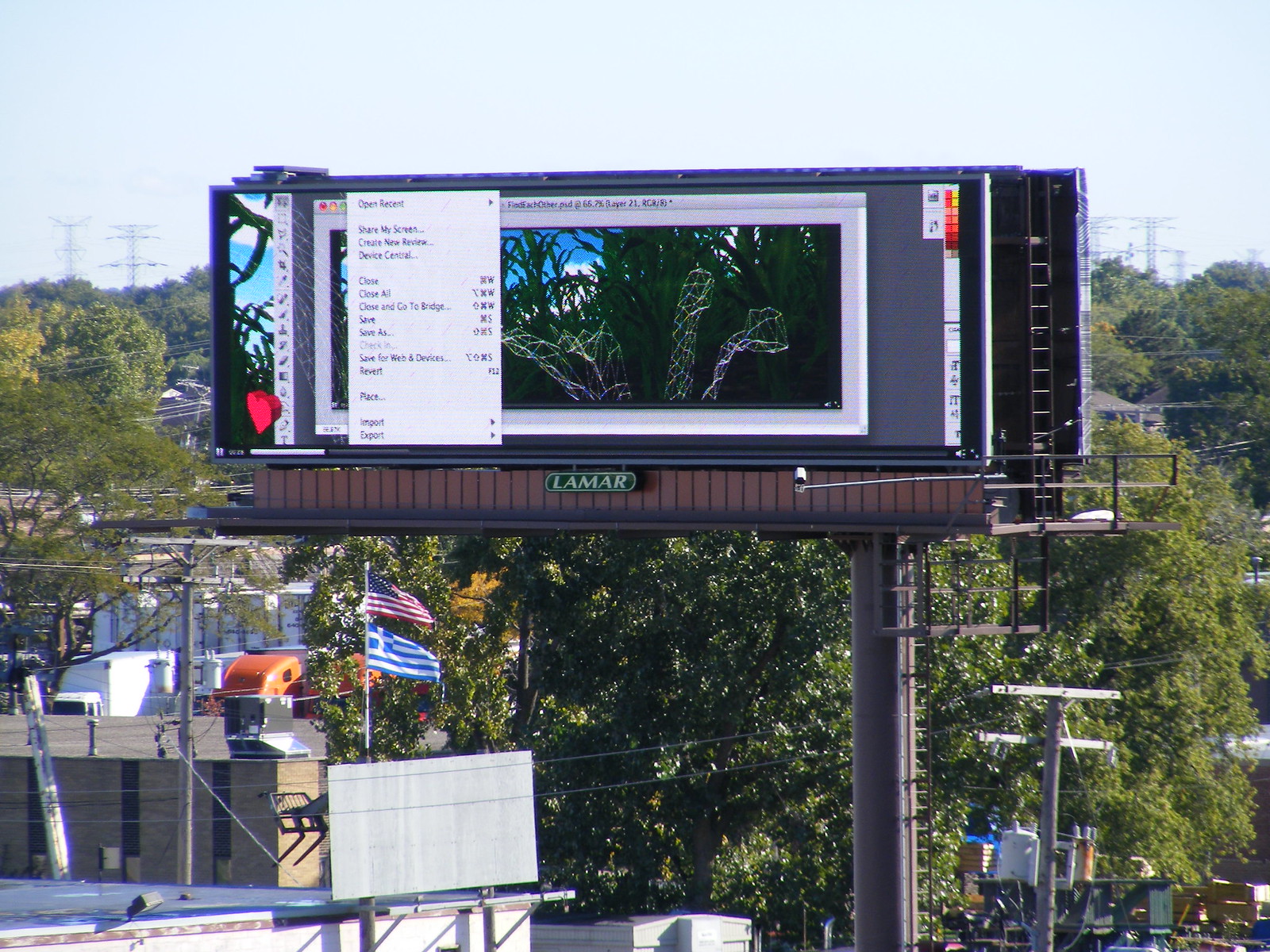The photograph captures a bustling outdoor scene featuring a high-standing billboard prominently set among rooftops, power lines, and telephone wires during the daytime. Erected on a sturdy brown wooden platform, the billboard is flanked by a flagpole displaying the United States flag at the top, with the Greek flag fluttering below, characterized by horizontal blue and white stripes and a white cross on a blue field in the upper corner. In the background, treetops and various industrial structures add to the busy atmosphere.

The billboard itself appears to be an electronic display showcasing a digitized screenshot of a computer screen. This screen features a drop-down menu on the left-hand side listing text such as "Open Recent" and "Clear All," along with iconic red, yellow, and blue buttons commonly found on a Macintosh interface for window controls. The main display area of the billboard shows a gray frame encasing a computer-generated image of vegetation, which includes leaves and possible tree illustrations against a bright blue sky, hinting at a work-in-progress setup for the digital content. The lower portion of the billboard platform bears a wooden brown paneled area with a visible Lamar logo, adding to the structured industrial aesthetic of the scene.